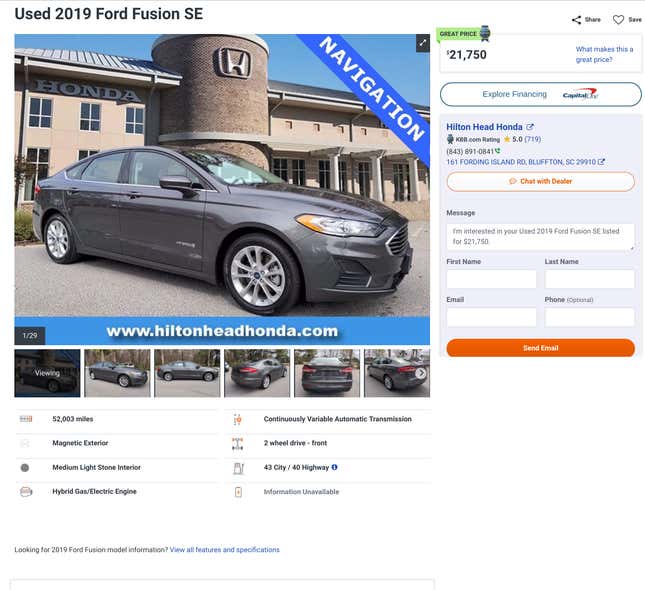Screenshot of a website featuring a car for sale: The website has a white background with the title "Used 2019 Ford Fusion SE" written in black at the top left. Below the title is a large photo of a gray, four-door sedan with chrome wheels, taken at an angle from slightly in front of the front tire, displaying the side of the car. The car is parked in front of a two-story Honda dealership with a prominent brick column in the center, displaying the Honda logo at the top.

Below the photo, a blue footer displays the website URL, www.HiltonHeadHonda.com, in white text. To the right of the photo, the price is listed as $21,750 with a green "Great Price" sticker above it. Below this, there is a button labeled "Explore Financing" featuring the Capital One logo. The section mentions "Hilton Honda," provides dealer ratings, a phone number, and a "Chat with Dealer" button. A form is available for prospective buyers to fill out their first and last name, email, and phone number.

To the left of the main photo, additional screenshots of the car are displayed along with a detailed list of the car's features.